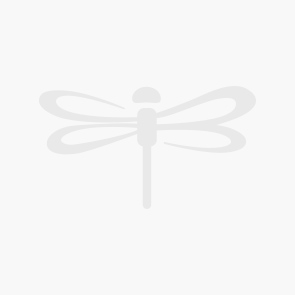This image is a detailed illustration of a simple, yet charming bouquet of flowers on a plain white background. The artwork features a variety of flowers, including two pink daisies with orangish-yellow centers and two purplish-blue violets with yellow centers. Additionally, there are three puffball-like flowers with an orange and yellow reflective texture, positioned in the top left of the bouquet. Small sprigs of lavender add a delicate touch to the overall arrangement.

The bouquet is tied together with a pinkish-red ribbon bow at the base, securing several long, slender green leaves that extend vertically. The leaves come in three shades of green: light green, dark green, and a muted, almost navy green. The illustration has a gentle texture, suggesting it might be hand-drawn, possibly on watercolor paper. The soft colors used in the artwork lend it a childlike, whimsical quality reminiscent of an illustrated children's book.